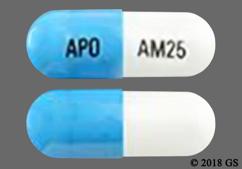The image features a grainy and compressed screenshot of a medical capsule displayed against a simple gray background. The capsule is shown in two views: the front and the back. The pill is divided into two parts: the larger outer half, which is a light sky blue color with "APO" printed in black uppercase letters on it, and the smaller inner half, printed with "AM 25" in black letters at a slight angle. In the bottom right-hand corner of the image, there is a copyright symbol followed by "2018 GS" in black text. The bottom view of the capsule reveals a seamless continuation of the pill with no additional markings. This image likely originates from a drug identification website, designed to help users cross-check and verify medications based on printed identifiers.